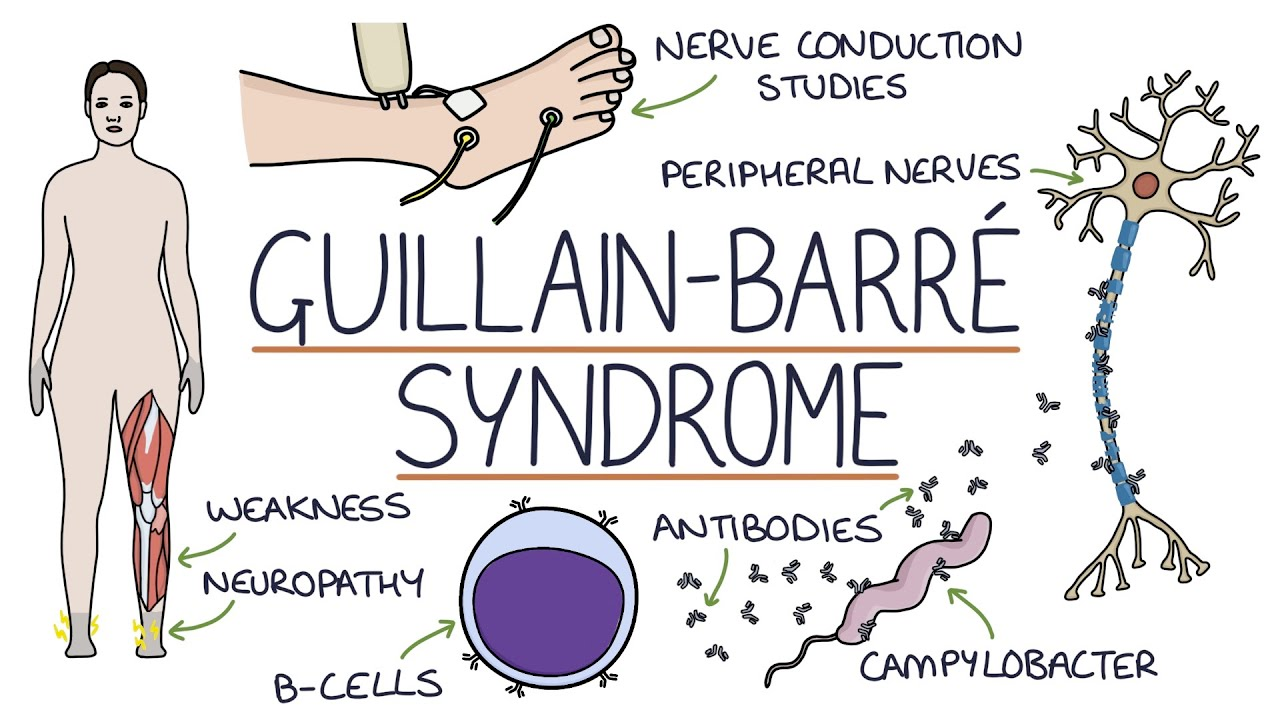This detailed infographic illustrates various aspects of Guillain-Barré Syndrome. Central to the image are large letters labeling the syndrome as "Guillain-Barré Syndrome." Around the central label, the infographic is populated with several smaller, cartoon-style images and labels, each highlighting distinct symptoms and biological components associated with the syndrome.

On the left side, a scientific illustration of a person is depicted with emphasis on the legs, showing internal muscle and bone structures. Labels point to this illustration, noting "Weakness" and "Neuropathy." The feet of the person are tinted gray, with lightning bolt symbols indicating severe discomfort or pain.

At the top of the infographic, an image of a foot with leads attached to it is shown, representing "Nerve Conduction Studies," a diagnostic test for nerve function.

On the right, a detailed illustration of a nerve cell, labeled "Peripheral Nerves," visually explains the syndrome's impact on the nervous system.

The bottom part of the infographic showcases several biological elements critical to understanding Guillain-Barré Syndrome. A round cell with differently colored intracellular components is labeled "B-Cells," and smaller structures attached to it are identified as "Antibodies." Additionally, a squiggly, worm-like figure labeled "Campylobacter" is depicted, indicating the potential bacterial trigger for the syndrome.

Overall, this infographic provides a comprehensive visual summary of the key features and diagnostic elements of Guillain-Barré Syndrome, integrating detailed annotations and clear, illustrative imagery.